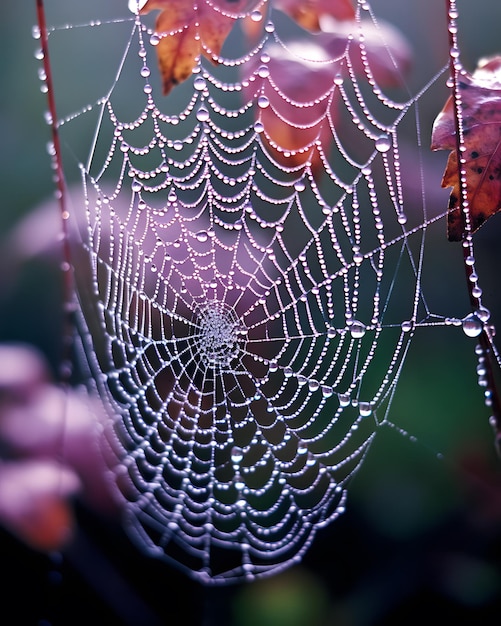This is a very close-up photograph of a spiderweb, showcasing its intricate beauty as it hangs suspended in the air. The web, which is completely intact, is adorned with hundreds of dewdrops, ranging in size from tiny beads to larger spheres. These droplets create a mesmerizing design, weighing down the web and causing it to sag slightly in some places. In the out-of-focus background, there is a rich tapestry of natural elements, including vibrant pink and red leaves, potentially flowers, and abundant greenery. The scene gives the impression of a forest setting, possibly in the fall, with the web attached to two slender branches. Notably, in the top right corner, there are a couple of red leaves speckled with black dots. The combination of the vivid spiderweb and the blurred backdrop highlights the delicate, shimmering structure of the web against the subtle hues of the surrounding foliage.